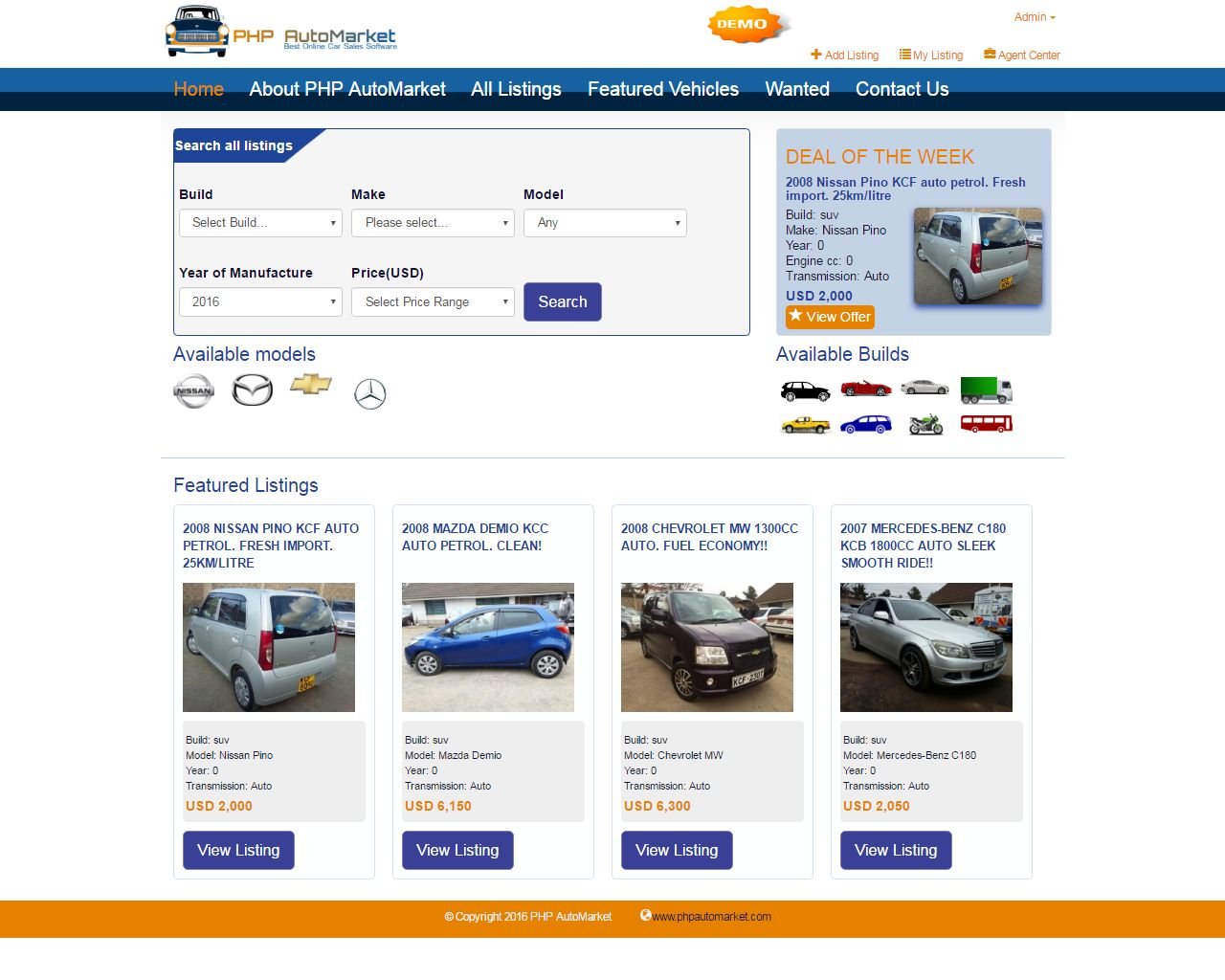The image depicts the homepage of a website named "PHP AutoMarkets," prominently displayed in blue text at the top left corner. Adjacent to its right is an orange logo labeled “Demo,” followed by a small “Admin” text. Just below, a navigation bar stretches across the screen, its background split into a blue top half and a black bottom half. 

The navigation items are listed as follows from left to right: "Home" in orange, followed by "About PHP AutoMarkets," "All Listings," "Featured Vehicles," "Wanted," and "Contact Us," all in white text. Beneath the navigation bar, a light gray search rectangle offers various filtering options including "Build," "Make," "Model," "Type of Manufacturer," and "Price," accompanied by a blue search button.

To the right side of this search section, there is a prominent "Deal of the Week" highlight, showcasing a 2008 Nissan Pino. The "Deal of the Week" text is in orange, and below it is blue and black text with an image of the vehicle.

Further down the page, the "Available Models," "Available Builds," and "Featured Listings" sections are displayed, featuring four cars. Each car listing includes the vehicle's name in blue text, an image of the vehicle, and the pricing in orange text. Every listing also has a blue rectangle at the bottom labeled "View Listing."

The footer of the image is marked by an orange bar that runs horizontally across the page, and the majority of the background remains white.